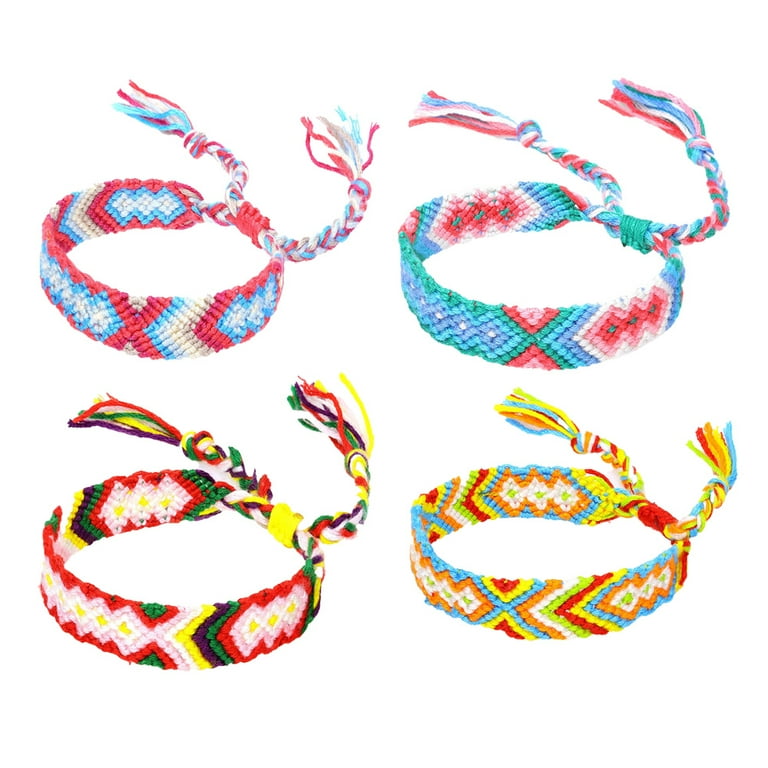This is a photograph of four intricately crafted headbands, each featuring a unique color palette and beaded design. Arranged in two rows of two on a white background, these accessories exhibit an exquisite sense of craftsmanship and detail. 

The upper left headband is adorned in red, white, and blue beads, presenting a vibrant and patriotic theme. Next to it, on the upper right, is a headband that has a turquoise blue base accented with bursts of white, red, pink, and a hint of green. Both of these headbands showcase a consistent beaded design, featuring thick, intricately beaded bands that taper into smaller straps for tying at the back.

On the lower left, the headband boasts a colorful blend of yellow, pink, red, and subtle green accents, forming a warm and lively composition. The bottom right headband is the most vivid of them all, with a lime green backdrop interwoven with red, light blue (or baby blue), and touches of orange, creating a bright and colorful appearance. 

Collectively, these headbands, with their detailed beaded work and colorful designs, suggest a possible Native American influence, although the specific tribe is unidentified.